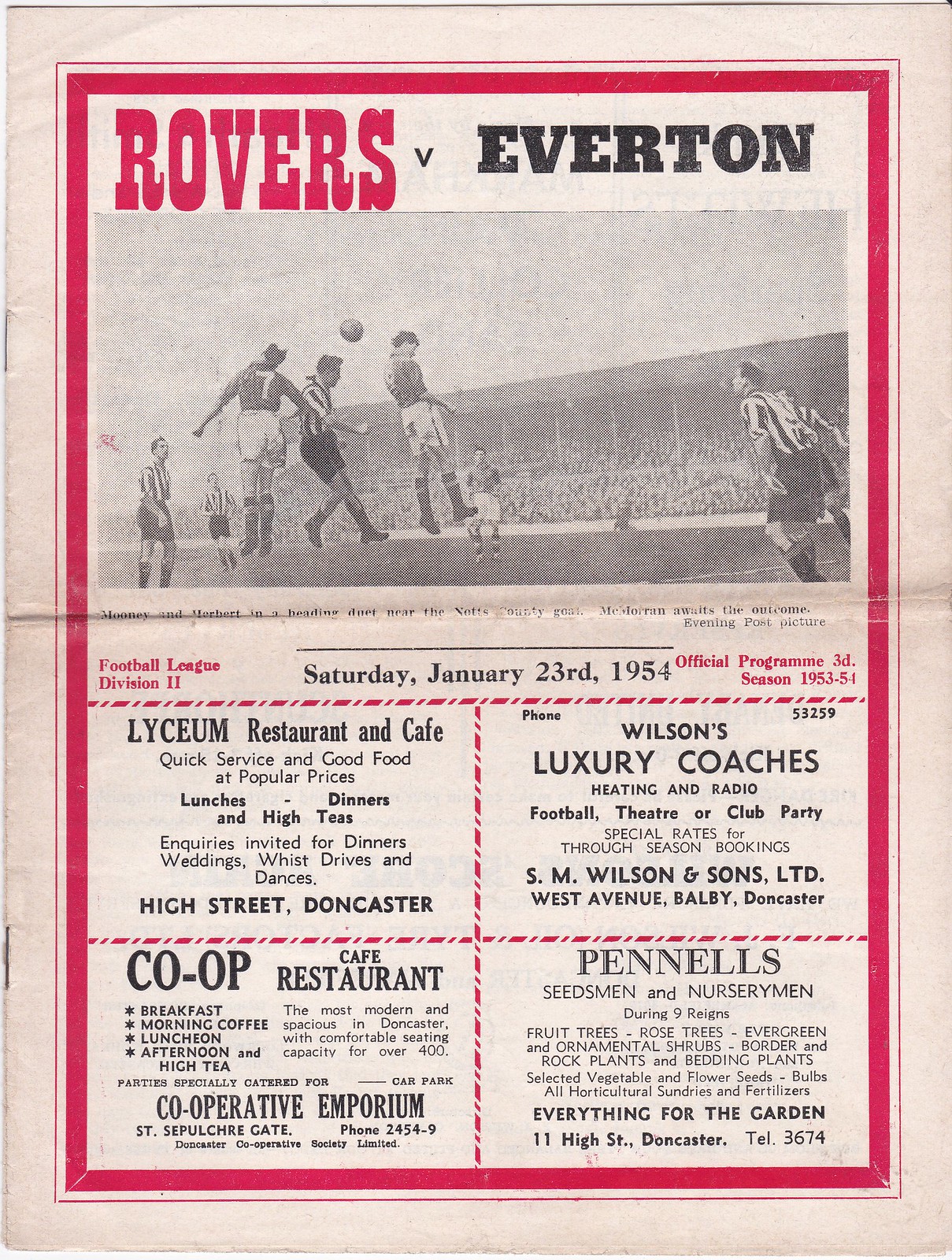The image depicts the distressed front cover of an old sports program, featuring a creamy-colored background, tanned from age, and a red border around the edge. The top of the page reads "Rovers vs. Everton" with 'Rovers' in red letters and 'Everton' in black. Below this title, there's a black-and-white action photograph of a football match, showing a scene where a player in a number seven shirt attempts to head the ball while another player in a black and white striped shirt challenges him. The description, "Mooney and Herbert in a heading duet near the Knotts County goal. McMoran awaits the outcome, evening post picture," is written in black text near the crease from the center fold.

The date, "Saturday, January 23rd, 1954," confirms the program's vintage, signifying it as the official program for the Rovers. Below the main image, the layout is divided into four rectangular advertisements, each bordered in red, promoting local businesses: Lyceum Restaurant and Cafe, Co-op Cafe Restaurant, Wilson's Luxury Coaches, and Pennell's Seed Men and Nursery Men. The page density and creases emphasize its historical context, hinting at its magazine origin filled with various sponsors' ads.